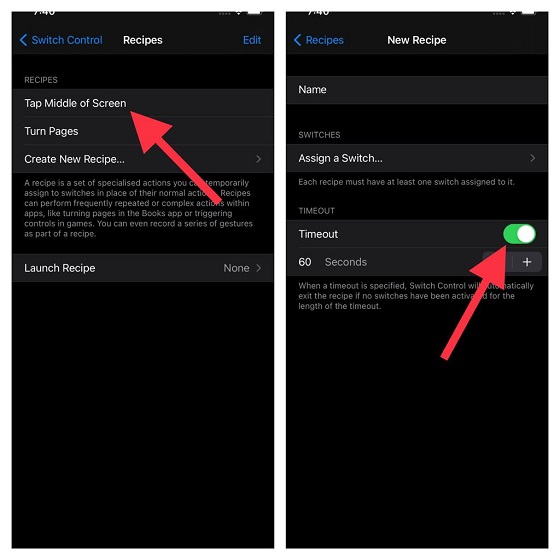In this image, we observe two side-by-side screenshots of a user interface, both set against solid black backgrounds, featuring blue and white text.

**Left Screenshot:**
- Displays a section titled "Switch Control" in blue text at the top.
- Directly below, it reads "Recipes" with an "Edit" button adjacent to it.
- A red edited arrow points to the "Recipes" section.
- Underneath, there's a navigational instruction: "Tap middle of screen."
- Below this instruction, it lists options: "Turn Pages" and "Create New Recipe."
    - Description for "Create New Recipe": "A recipe is a set of specialized actions you temporarily assign to switches, replacing their normal functions. Recipes can facilitate frequently repeated or complex actions within apps, like turning pages in the Books app or triggering controls in a game. You can even record a series of gestures as part of a recipe."
- Towards the bottom, it has a bolded white text option labeled "Launch Recipe."

**Right Screenshot:**
- Follows a similar visual format and layout as the left.
- The title reads "New Recipe."
- Below the title are the fields: "Name," "Assign a Switch," and "Timeout."
- The "Timeout" section includes a toggle switch that is turned on, set to 60 seconds.
- A red arrow, similar to the one in the previous screenshot, points to this toggle switch.

This detailed layout captures the process of creating a custom switch control recipe for specialized actions, aiding users in managing frequent or intricate tasks on their device.